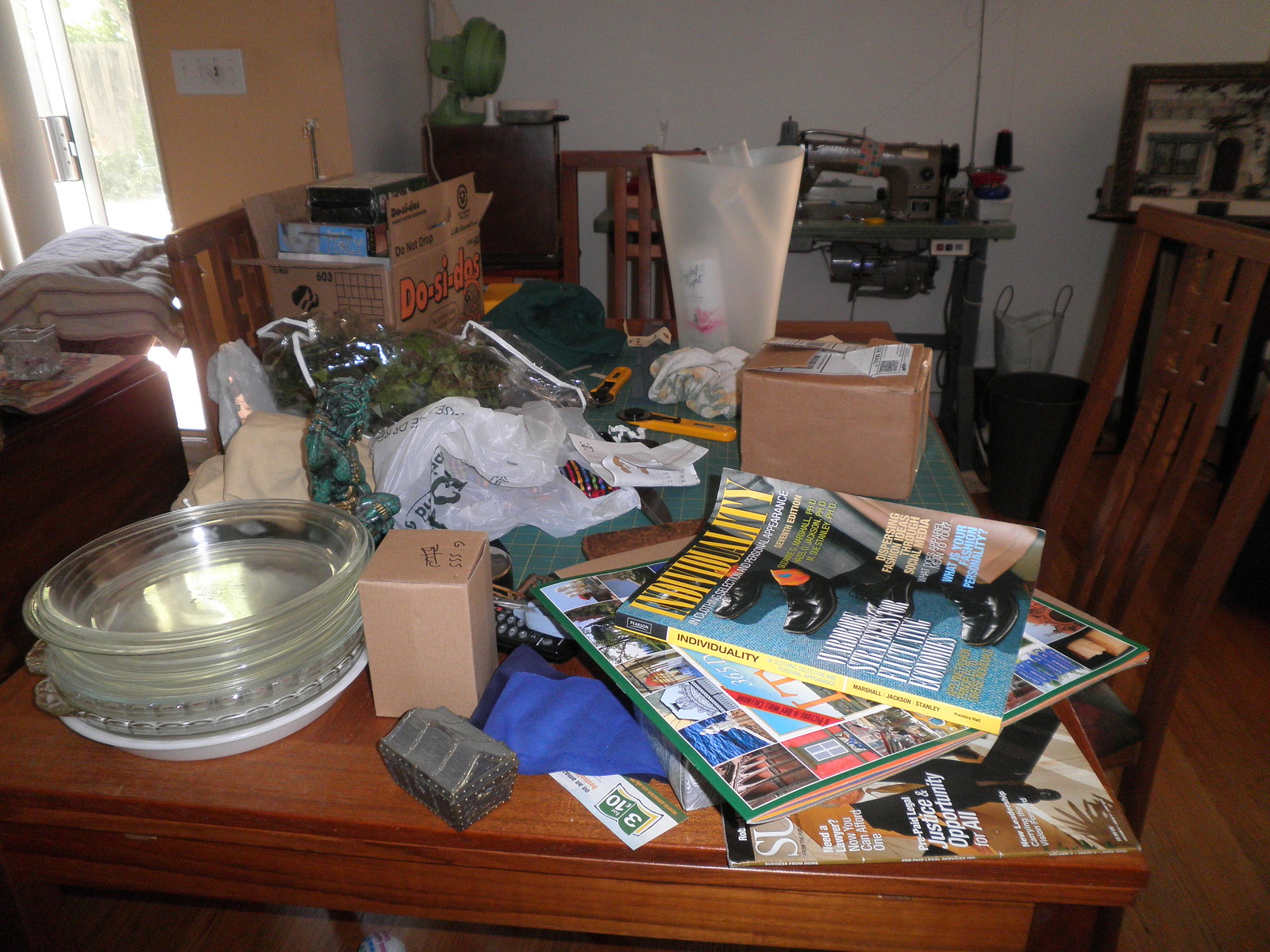This image depicts a large, square room inside a house with various elements and objects scattered throughout. Toward the back left, a sliding glass door with silver frames and vertical white blinds reveals a bright, sunny day outside, showcasing glimpses of green foliage, a brown patio, concrete, leaves, and trees. To the right, the backside of a large cabinet, bare with exposed particle board, is visible. Atop a brown surface sits a green fan.

The room appears to be a workspace or hobby area, as evidenced by several tools, such as sanders and circular saws, set against the white walls in the background. A framed picture decorates one of the walls. To the left, white blankets are neatly folded on an ottoman or couch cushion. Atop this cushion, there appears to be a book or glass cup.

The main focal point is a central table, cluttered with a plethora of items. Among these are several magazines, an Amazon box, another box labeled "Do-si-dos," and various other boxes nested inside. Shopping bags, pieces of fabric, small glass bowls, and what seems to be a coupon complete the chaotic yet intriguing scene, reflecting a space full of activity and daily life.